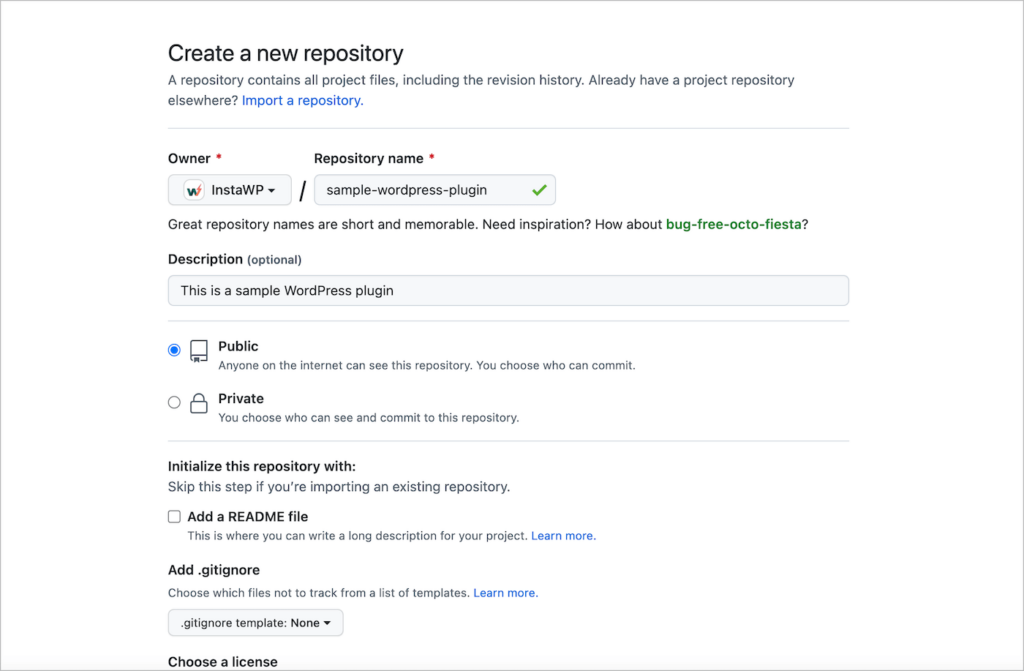The image depicts a screenshot of a web interface for creating a new GitHub repository. It consists of several sections and elements:

1. **Header**: A rectangle outlined in a thin black line with the text "Create a new repository." This panel introduces the purpose of the page, mentioning that a repository contains all project files including the revision history. It also provides an option in blue text to "Import a repository" from elsewhere.

2. **Form Fields**:
   - **Owner**: Labelled with an orange star, indicating it's a required field.
   - **Repository Name**: Also marked with an orange star, signifying it's mandatory.

3. **Repository Naming Suggestions**:
   - There's a section that encourages the creation of short and memorable repository names. It provides an example in green text: "bug-free Fiesta."

4. **Description**:
   - An optional field titled "Description" with a blue rectangle containing the sample text "This is a sample WordPress plug-in."

5. **Visibility Options**:
   - **Public**: Represented by a blue circle with an image of a screen and some unreadable text.
   - **Private**: Indicated by a gray outline circle with a lock icon and additional unreadable text.

6. **Initialization Options**:
   - A gray outlined square with "Add README file," accompanied by some unreadable words, the last two of which are in blue.
   - Another section for "Add .gitignore," also containing unreadable words with the last two in blue.
   - An option for "Choose a license," albeit with some words not fully visible.

7. **Graphics and Logos**:
   - A blue-gray rectangle featuring a white circle with a split-color 'W' (part blue, part orange) and the text "InstaWP" with a downward-pointing arrow.
   - Another gray rectangle titled "sample-WordPress-plug-in" followed by a green check mark.

The entire setup is aimed at guiding the user through the process of setting up a new repository with various customization options and helpful hints.

**Note**: Some text and elements in the image are too small to read clearly.